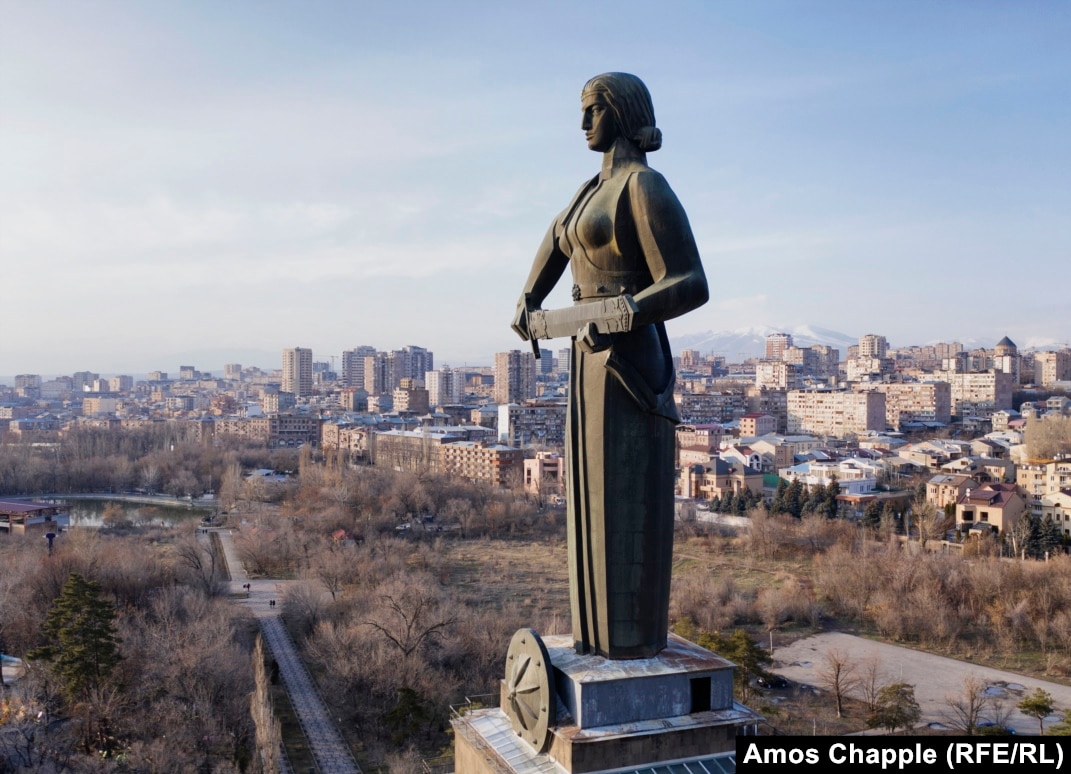A majestic iron statue of an imposing woman stands prominently against a panoramic city skyline. The statue captures her left profile as she gazes sternly towards the left, her short hair trailing behind her head. Her muscular, angular arms grip a large sword just above her waist, with the handle held firmly in her right hand and the blade in her left. The woman is dressed in a long, straight gown that conceals her feet, and her round breasts are defined just above the upper torso. Positioned on a square platform, the statue also features a green-colored shield mounted in front. The city's skyline, full of towering skyscrapers and assorted buildings of varying sizes, stretches out behind her. A roadway meanders through barren trees towards a body of water on the left, suggesting a chilly, winter-like season. Below the statue and in front of the cityscape is a park with dead grass and bare trees, accentuating the wintery feel. In the bottom right corner of the image, it reads "Amos Chapel (RFE/RL)." The overall scene conveys an aura of strength and monumentality, set against an expansive urban backdrop and a distant snow-capped mountain.